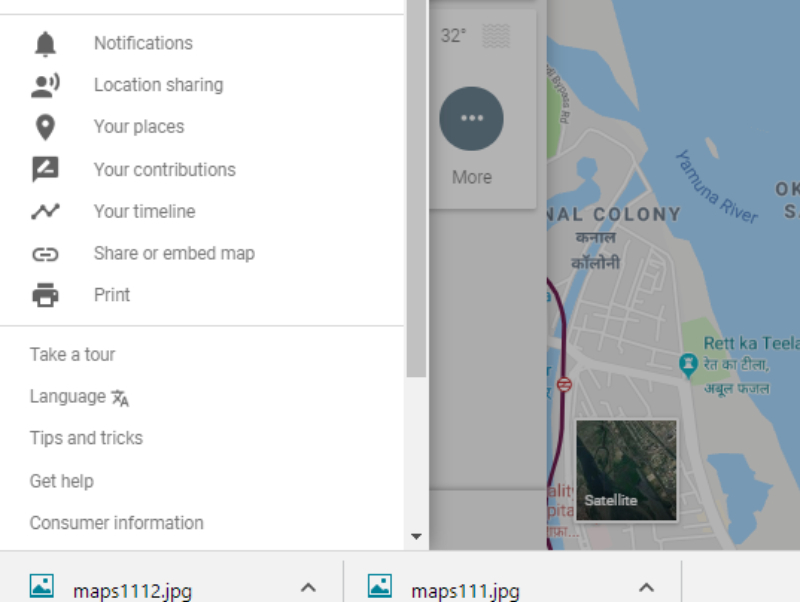Screenshot of a computer screen displaying a Google Maps interface with various features and notifications. On the left side, small gray icons are visible for functions such as notifications, location sharing, your places, your contributions, and an embed map. There are also options to take a tour, change the language, and access tips and tricks. A scroll bar is shown on the right.

Prominently displayed is a weather overlay on the map, which appears to be focused on a region in Asia. Satellite imagery is clearly visible within the map pane. At the bottom of the screen, two downloaded map files named "maps1112.jpg" and "maps111.jpg" are shown, each with a photo icon and an upward-pointing arrow next to them, indicating additional actions available for these files.